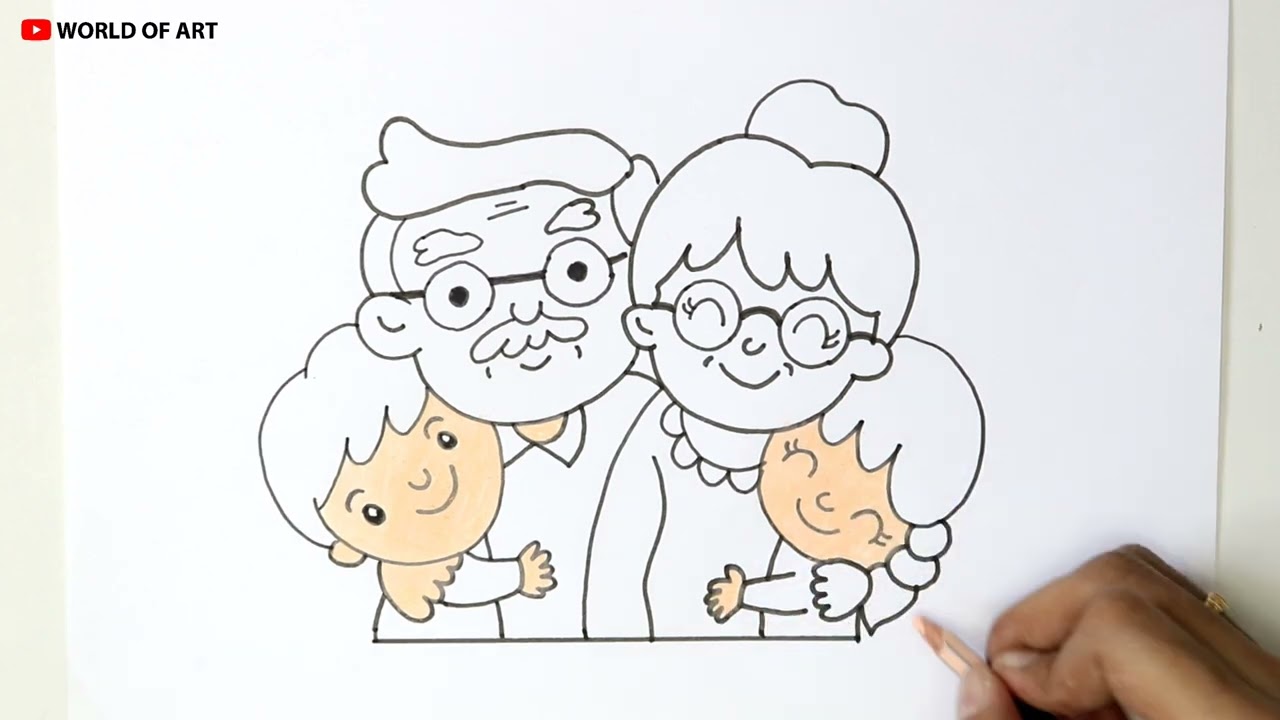In the image, a person's hand, adorned with a ring, holds a peach-colored pencil, actively coloring a detailed family drawing on a white piece of paper placed on a white table. The drawing depicts a joyous scene with a grandfather and grandmother, both wearing glasses, accompanied by their grandchildren, a boy and a girl. The grandfather, with a mustache, has open eyes and is smiling, holding the boy who also has a smiling face. The grandmother, with her hair tied up in a bun, is hugging the girl, and both have their eyes closed, sharing a tender moment. The person coloring has started filling in the skin tones for the children's faces and hands, the grandfather's hand and neck, and the child's ear on the left. The entire setting is shown against a cream-colored wall. In the top left corner of the image, there is a YouTube logo accompanied by the text "World of Art," indicating this is likely a screenshot from an art tutorial video.